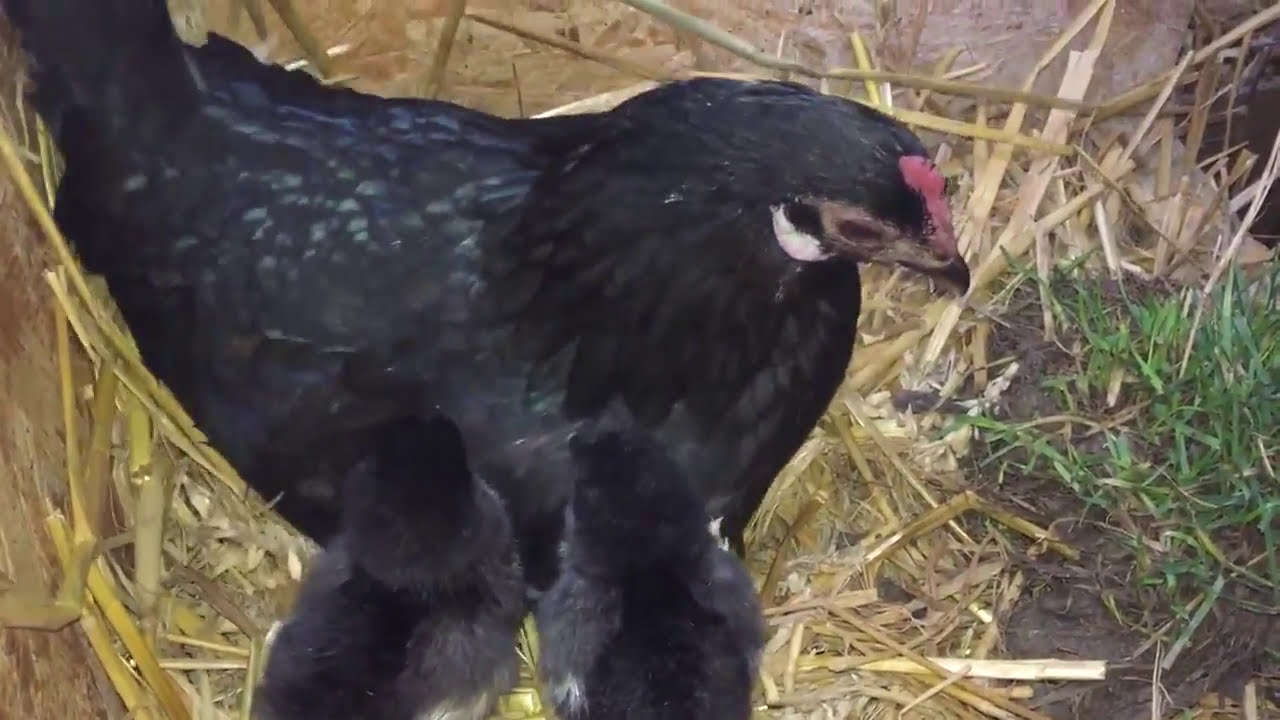In the close-up image, a large black hen with a red comb and white feathers on her neck is prominently featured. She is seated on a bed of yellow hay, with tufts of green grass peeking through on the right side. The hen's brown eye is partially visible as she gazes downward, seemingly over her two young, black and gray chicks who are nestled closely beside her, though their faces are not visible. The chicks, noticeably smaller and wingless, appear to be nestling in the hay near their mother. The background is filled with straw of varying lengths, and a tan-colored wall can be seen at the top of the image, adding to the rustic, farm-like setting.